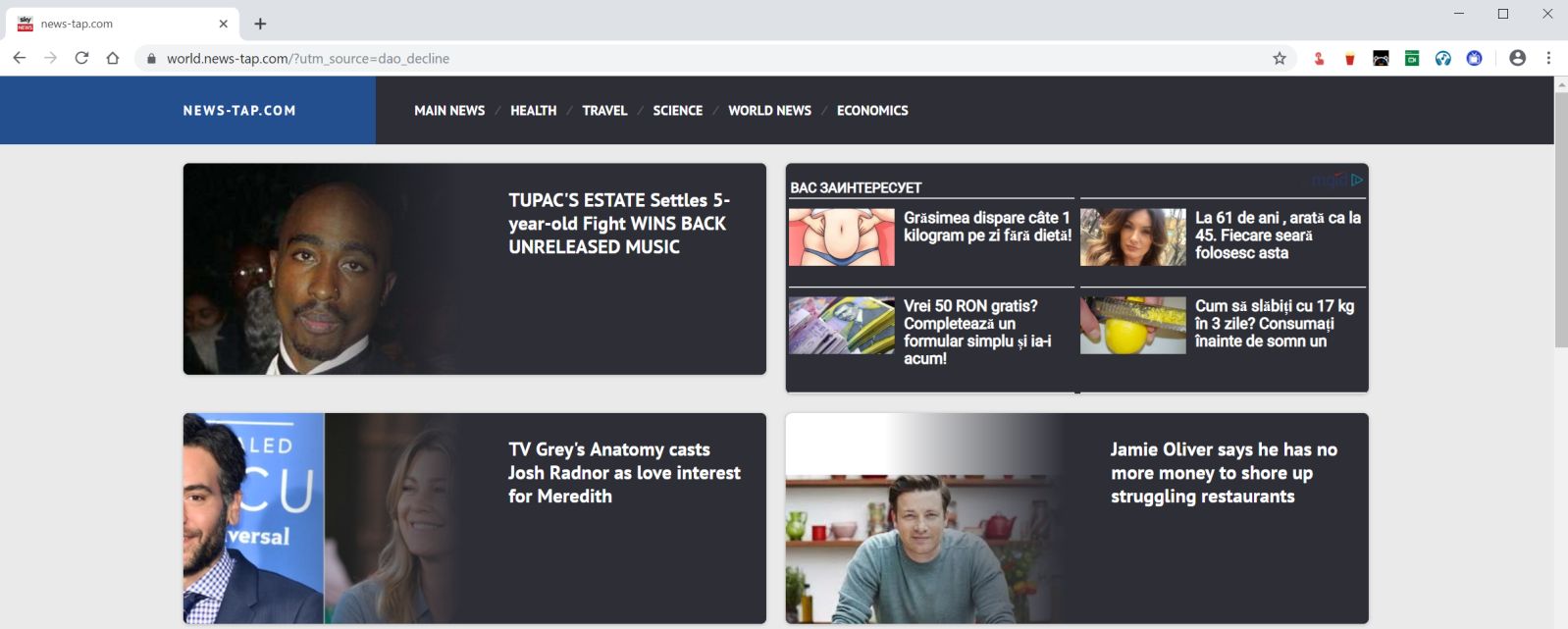The provided image depicts the landing page of the website "WorldNewsTap.com," which features a challenging-to-read top section. The URL, partially visible, is "worldnewstap.com." A prominent banner at the top of the page displays the website's name, "newsTap.com," along with several navigation options, including Main News, Health, Travel, Science, World News, and Economics.

The leftmost one-fifth of the banner is highlighted in a darker blue with "news tap" emphasized on it, while the other navigation options are displayed on a black banner spanning the width of the page.

Below the banner, four major stories are listed. In the top left quadrant, there's a headline that reads, "Tupac's estate settles five-year-old fight, wins back and releases music." To the right, there is another headline in French, featuring four bullet points that appear to be unclear, thereby causing some understanding issues.

In the lower left-hand corner, a story about television's "greatest Academy cast" highlights Josh Radnor as a love interest opposite Meredith. In the bottom right-hand corner, there's a headline regarding Jamie Oliver, stating that he has no more funds to support his struggling restaurants, indicating financial difficulties.